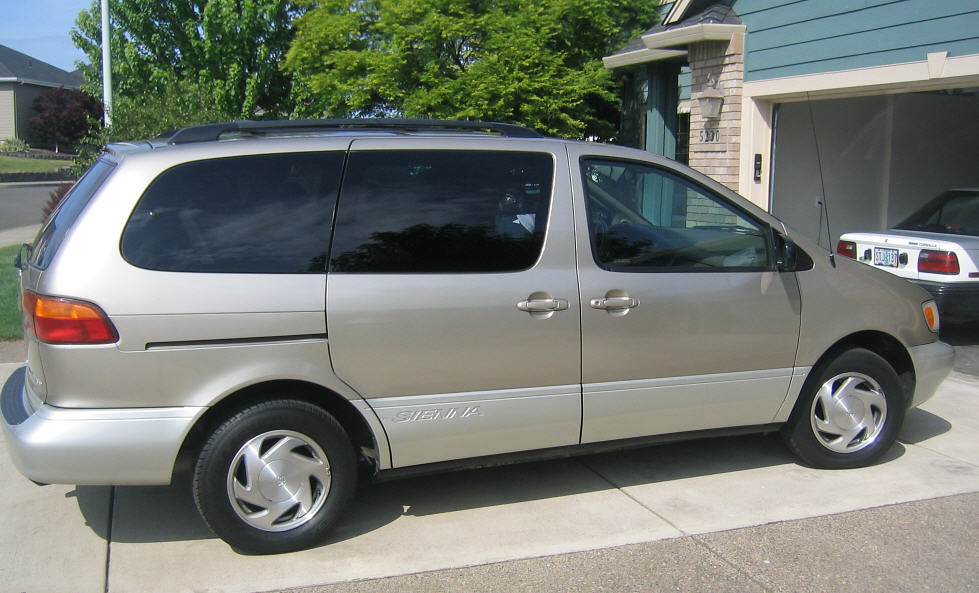The image shows a color photograph of a light gold Toyota Sienna minivan parked in a cement driveway in front of a blue and brick facade house. The minivan, featuring blackened rear windows, black tires with silver rims, and a roof rack, faces toward an open garage where a small white Toyota Corolla is parked. Above the house number 5230, a light fixture is visible. The daytime setting is underscored by a blue sky visible in the upper left corner. In the background, some trees and another house across the street can also be seen, adding to the neighborhood atmosphere.